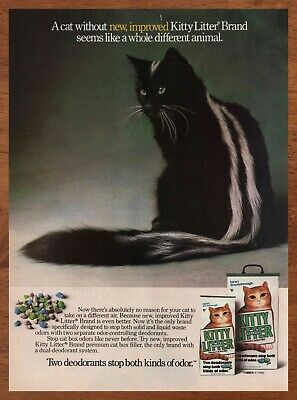This vintage magazine advertisement for kitty litter features a striking image of a black cat spray-painted to resemble a skunk, complete with two white stripes extending from its head, down its back, and along its tail. The cat is sitting on a white table, set against a dark grayish-black background, giving the visual a dramatic contrast. Encasing the whole ad is a thin brown wooden-looking border. The prominent text at the top reads, "A cat without new improved kitty litter brand seems like a whole different animal." The lower part of the page showcases two different-sized packages of the kitty litter, one with a black handle, both labeled with an orange tabby cat and green text. On the bottom left corner, a small image displays the granule texture of the kitty litter, described as green and black stones. Additionally, the slogan at the bottom declares, "Two deodorants stop both kinds of odor." The detailed design emphasizes the product's odor-fighting capabilities and distinct looks, aiming to capture the reader’s attention with its unique visual metaphor.